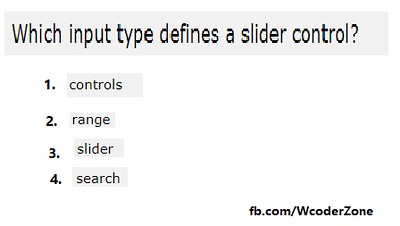An image is primarily white with sparse black text. Central to the composition, a question is posed: "Which input type defines a slider control?" Four options are provided beneath this inquiry:

1. controls
2. range
3. slider
4. search

The question and answer choices are presented in a blocky font that suggests a distressed, ink-depleted look. In the bottom right-hand corner of the image, the text "FB.com/WcoderZone" appears in a bold, Impact-type font, standing out due to its heavy, solid lettering. The image is stark, featuring nothing beyond the text and the plain white background, creating a minimalist and straightforward visual experience.